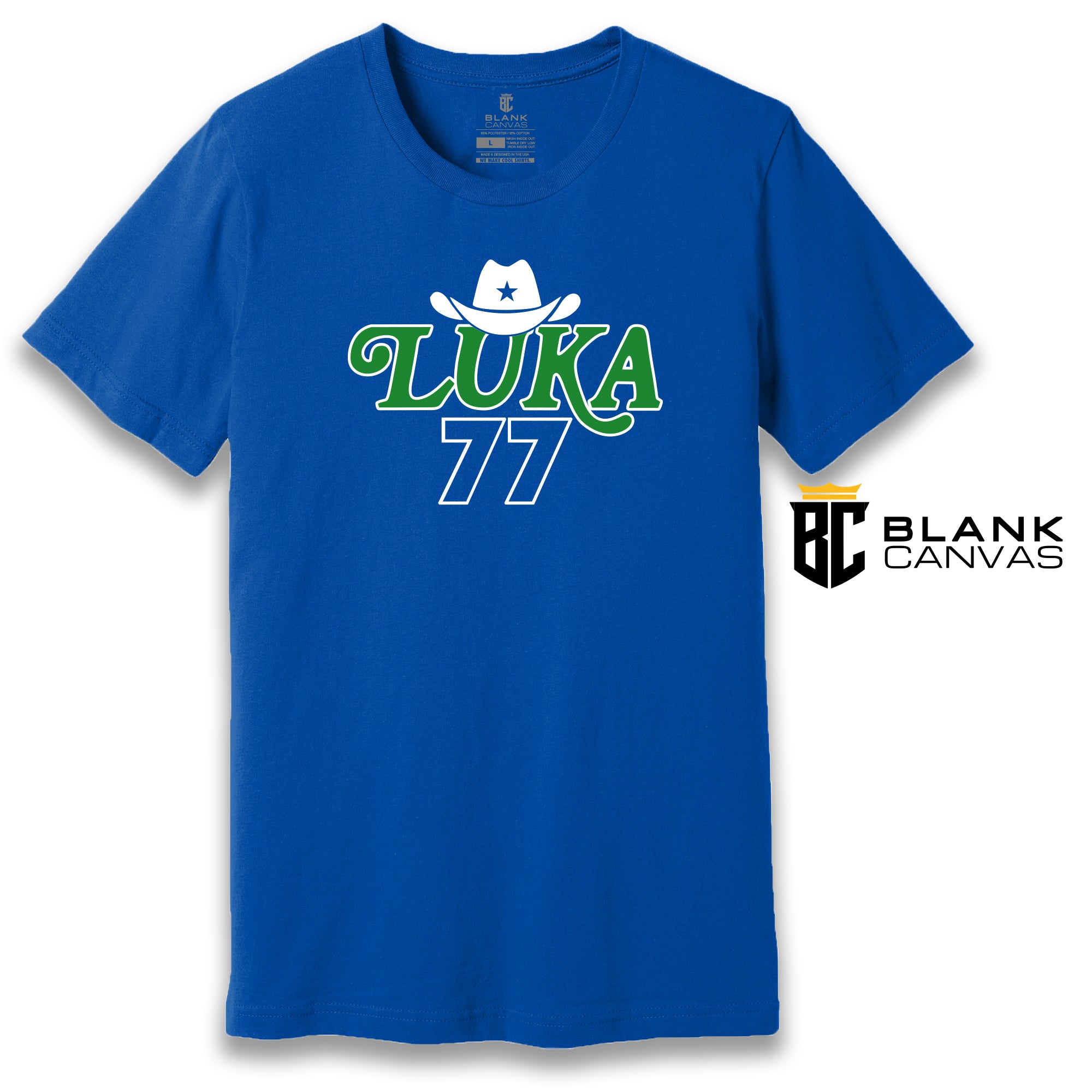A vibrant t-shirt designed for Dallas Mavericks fans, featuring the team's signature blue and green colors. The shirt prominently displays the number 77, symbolizing the superstar Luka Dončić, along with his name, making it a must-have for any dedicated fan. The design includes a cowboy hat decorated with a star, adding a touch of Texan spirit. Created by BC Canvas, also known as Blank Canvas, this short-sleeved tee offers comfort with its tagless design and lightweight material. Although Luka himself couldn't possibly wear it, this well-crafted shirt allows supporters to proudly show their love for the player during games or casual outings.